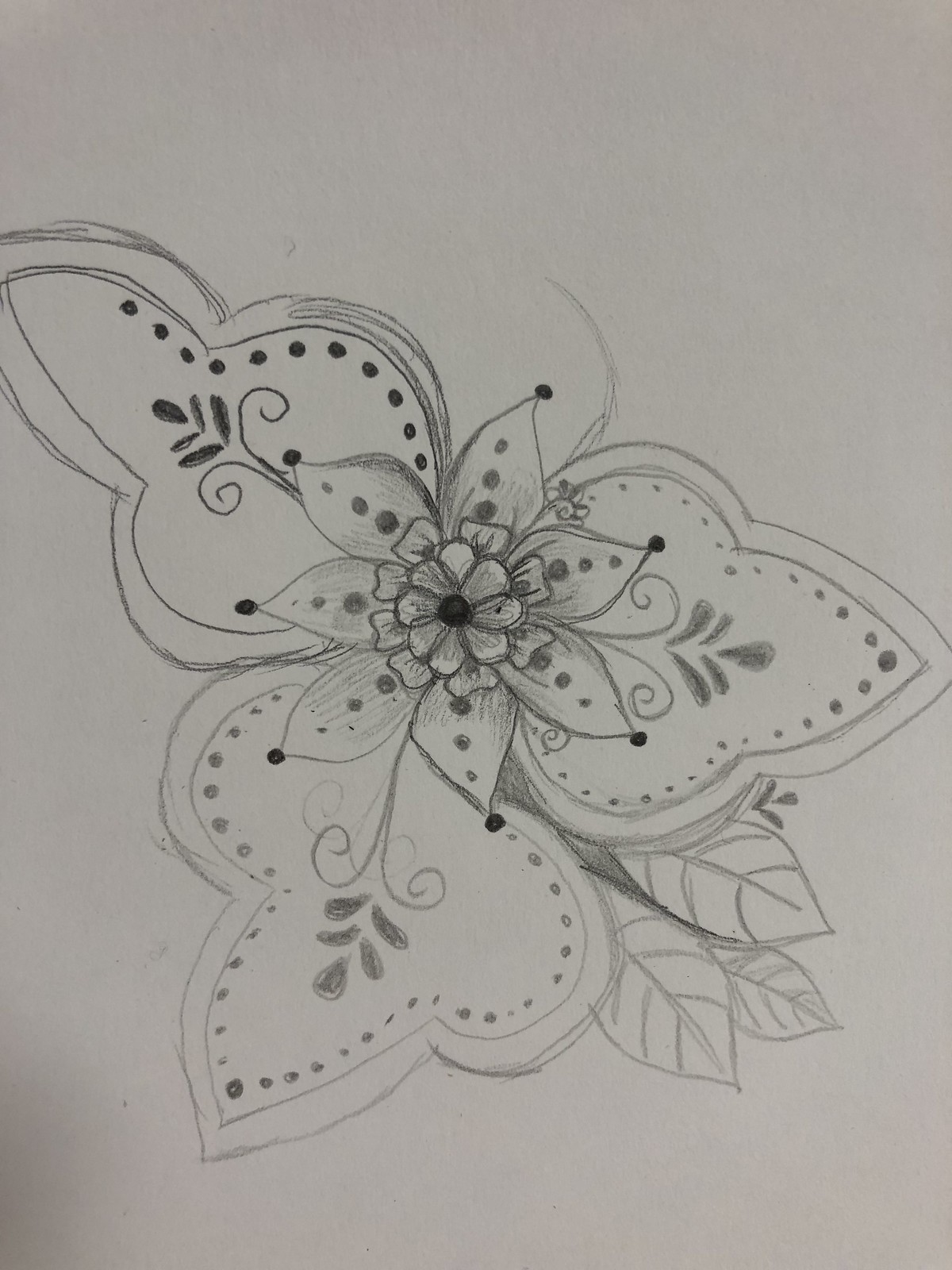This intricate drawing, crafted in pencil or pen on a pristine white background, showcases an elegant floral design that could be suited for embroidery, lace making, or purely as an engaging artistic sketch. The composition features three lobed leaves, adorned with delicate dots along their inner edges and accentuated with lines that emphasize their truffle-like shapes. Each leaf hosts a graceful scroll in its center. Dominating the heart of the design is a large, open flower with seven outer petals, encircling a ring of inner petals, and another central ring, contributing to its layered complexity. The arrangement exudes an appealing symmetry and fluidity. Complementing the main elements, two small leaves extend from the right-hand side, adding a final touch of balance to this pleasing pattern.